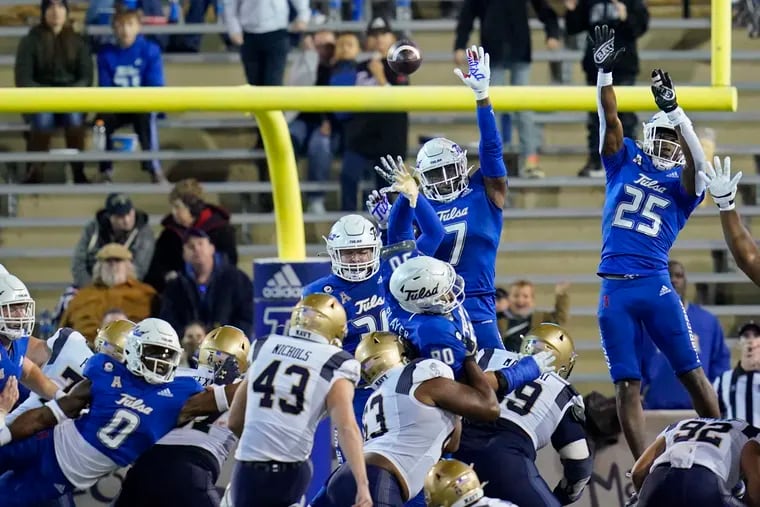In this detailed photograph of a college football game, we see a crucial moment near the field goal post, indicating a field goal attempt or extra point try. The action centers around two clashing teams: one in bright blue uniforms with white helmets and "Tulsa" emblazoned on their fronts, and the opposing team in white jerseys with dark blue pants and gold helmets. The Tulsa players are leaping with their hands raised in an attempt to block the flying football, which is visible just above their hands. The yellow goal post, padded with blue safety foam, stands prominently in the background. Behind the frenetic action, fans and families are visible on gray bleachers, bundled in jackets suggesting cold fall or winter weather. A referee, whistle in mouth, watches intently from the right side of the frame as the ball rises. The stands are not densely packed, offering a clear view of the decisive play happening on the field.